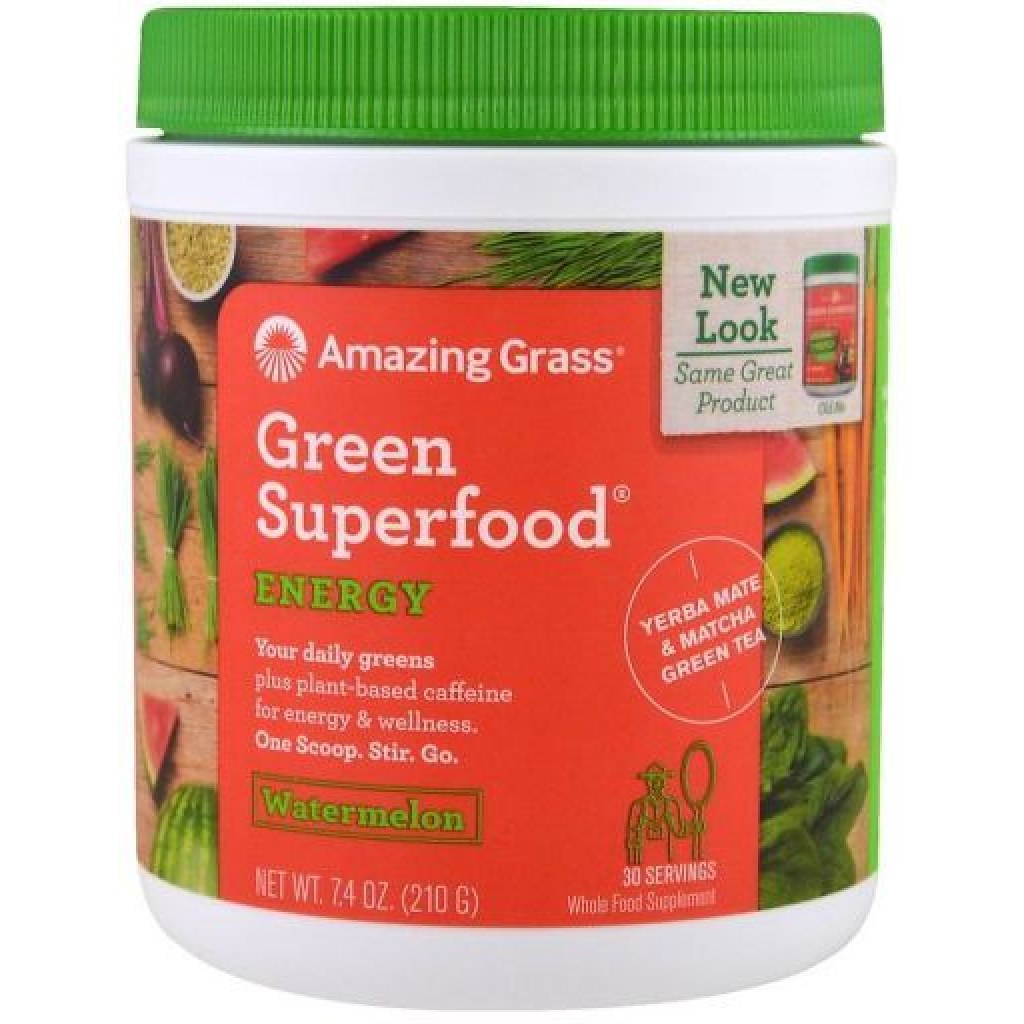This image features a white plastic jar adorned with a vibrant label, complemented by a green lid. The label prominently displays an array of colorful vegetables, enhancing its visual appeal. The brand name, "Amazing Grass," is boldly highlighted along with a product title: "Green Superfood Energy." The description on the label states that this supplement provides "your daily greens plus plant-based caffeine for energy and wellness." The usage instructions are succinct: "One scoop. Stir and go." Indicating its flavor, the jar is marked "Watermelon." Additionally, a logo at the bottom of the label specifies the jar contains "30 servings."